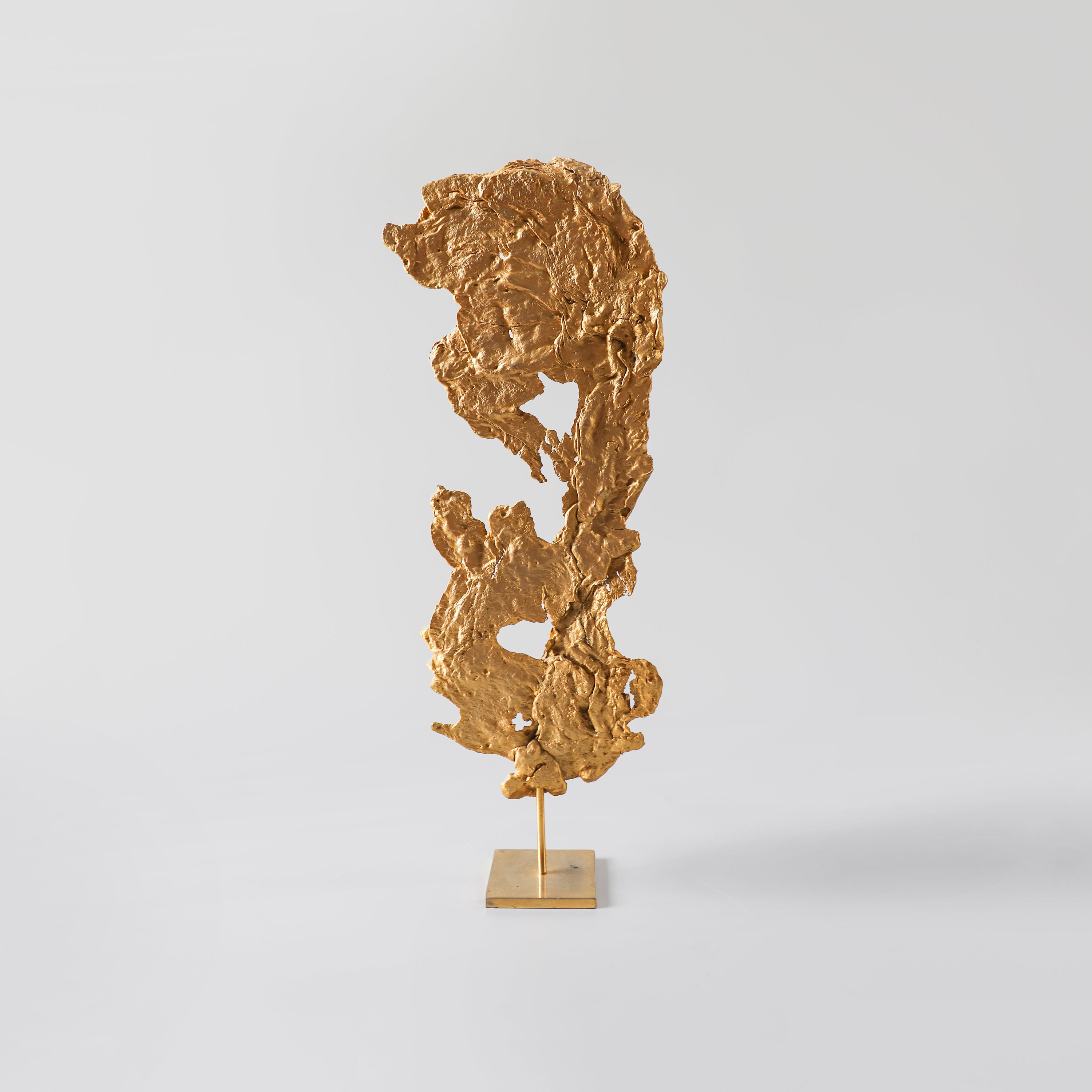The photograph showcases a gilded abstract sculpture by Philippe Chiverny, created around 1970, against a light gray background with a visible shadow stretching towards the bottom right. The vertically rectangular image, devoid of any borders, draws focus on the central sculpture mounted on a small golden square base. Rising from this base is a slender golden pole supporting the sculpture, which resembles a nugget of gold that has melted and dripped down, forming intertwined, undefined strands that twist and turn with no discernible pattern. The gilded artwork features open spaces at both the top and bottom, and its surface texture mimics that of a rock. The overall style is photographic representationalism, capturing the realism of this sculpted art piece.